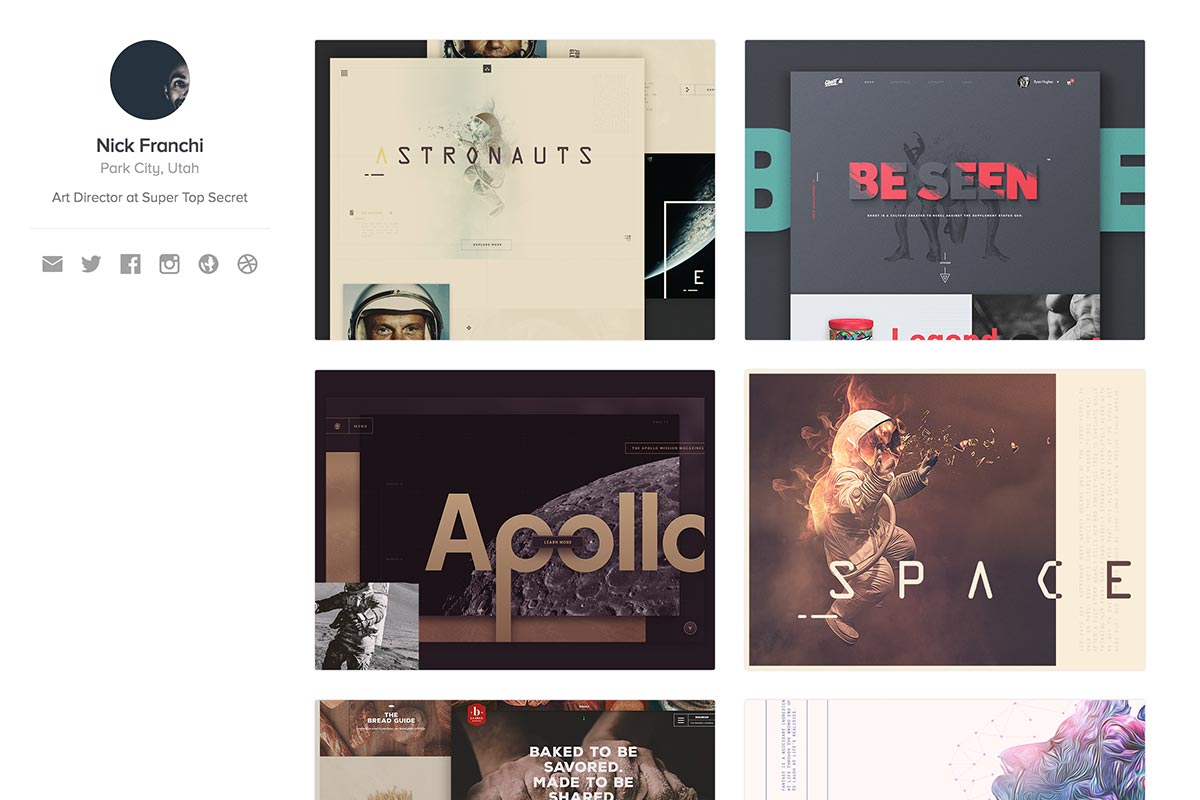Caption for the Image:

"Nick Franchi, an art director at Super Top Secret in Park City, Utah, is depicted in this artistic collage. The layout features a variety of symbols including an envelope, the Twitter bird, Facebook logo, and Instagram icon, alluding to modern communication and social media. Dominating the top left corner is a piece of artwork titled 'Astronauts' within a white square frame, portraying the adventurous spirit of space exploration. Central elements include a sphere that appears to be a basketball, juxtaposed with texts such as 'be seen' and 'Apollo,' emphasizing visibility and historic space missions. The image of the moon, complete with detailed craters, underscores the celestial theme. Interspersed throughout are stylized clouds, a brown background, and another phrase, 'Baked to be savored, made to be shared,' suggesting a fusion of communal enjoyment and artistry. Bottom right reveals a predominantly white section featuring a figure with distinct red strands framing their face, adding a human element to the cosmic narrative."